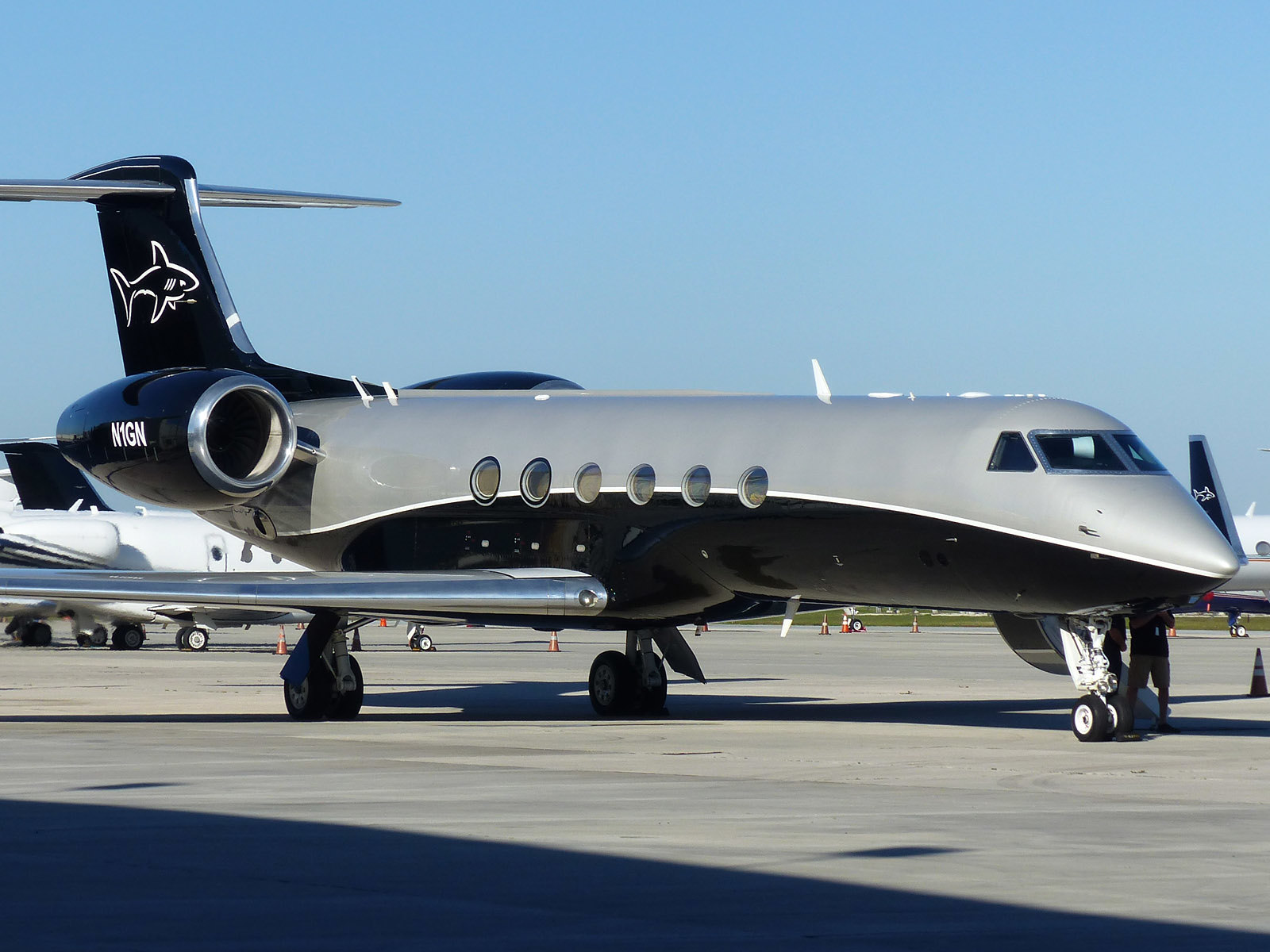The image captures a detailed scene at an airport runway under a perfectly clear, blue sky. Dominating the horizontal, framed photograph is a large, sleek airplane with a silver and dark blue exterior, pointed nose, and cockpit windows. The aircraft, which is positioned facing the right side of the picture, features six circular windows along its side and the registration number "N1GN" emblazoned in white on one of its engines. On the tail of the plane, a distinctive white logo depicts a dolphin. The wings of the plane extend upwards towards the top left corner of the image. A man stands underneath the nose of the airplane, adding a human element to the scene. In the background, partially visible are at least two other planes, appearing smaller due to the perspective. The runway showcases shadows of the planes, and a strip of grass can be seen faintly in the distance, complementing the overall atmosphere of the busy airport.